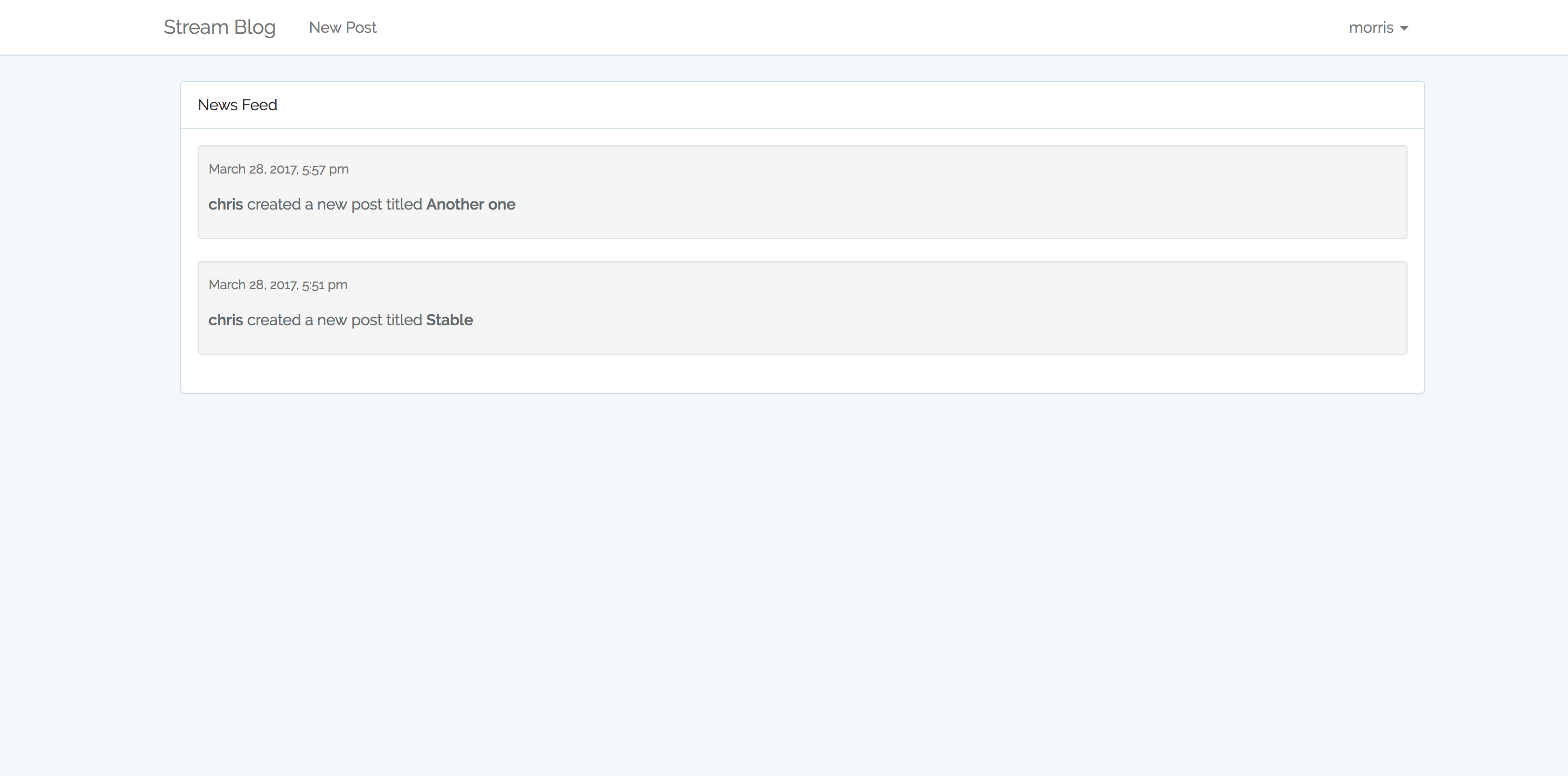The screenshot is of a blog interface. At the top left, in black text, it reads "STREAM BLOG." Beneath that, in a smaller font, it says "NEW POST." On the far right is a drop-down menu indicated by an arrow next to a name in small caps, "MORRIS," presumably referring to Morris' profile. All these elements are on a white strip at the top of the screen. 

Beneath this, the rest of the screen has a very light bluish-gray background. In the center, there is a text box with the heading "NEWS FEED" in black text. Below this, separated by a faint blue-gray line, are two entries contained in gray text boxes. 

The first entry states, "March 28th, 2017, at 5:57pm, Chris created a new post titled, ANOTHER ONE." The second entry reads, "March 28th, 2017, at 5:51pm, Chris created a new post titled, STABLE." This indicates that "STABLE" was the first post, followed by "ANOTHER ONE."